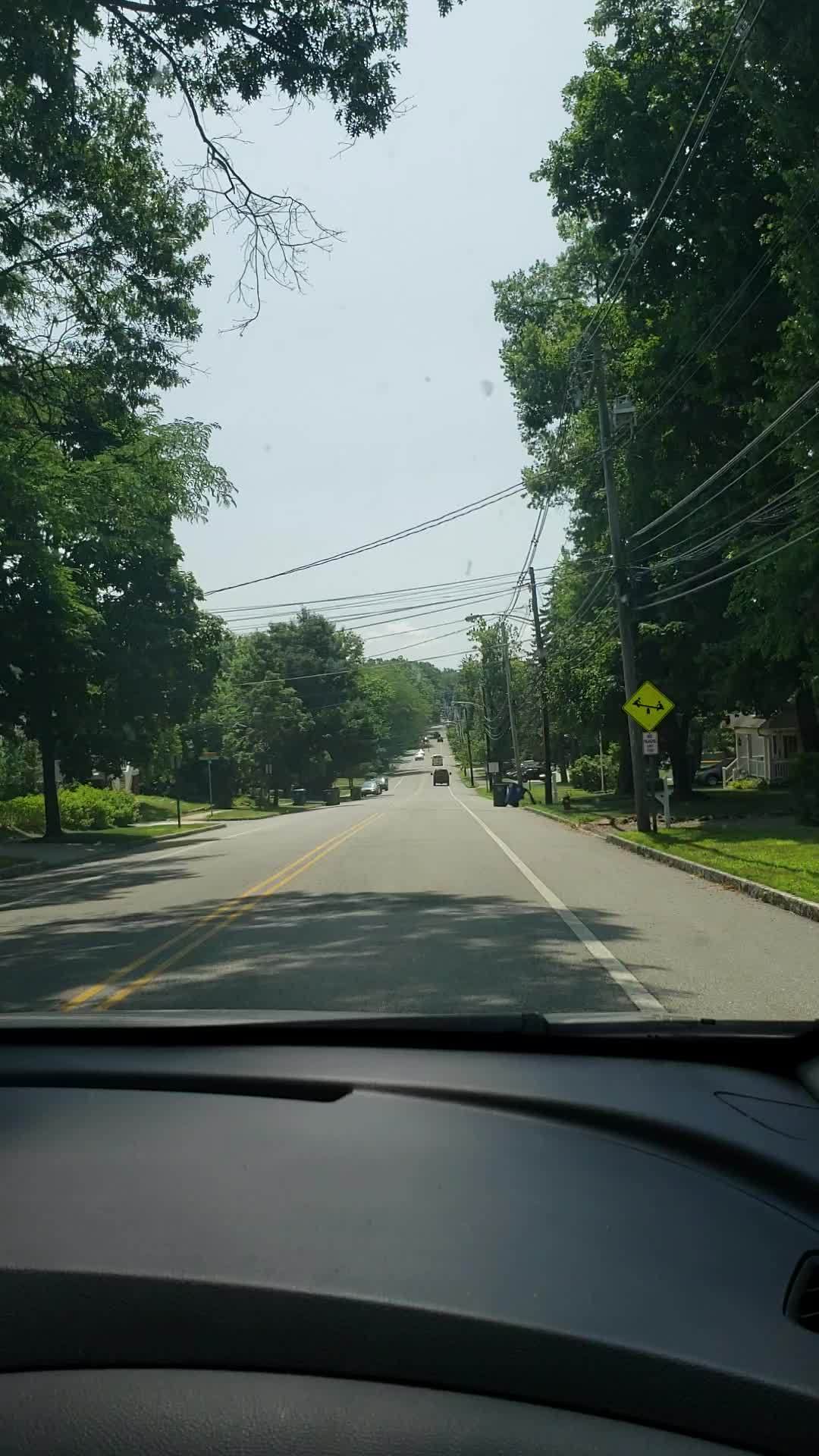A detailed photograph captured through the windshield of a car traveling on a road, showcases a vibrant street scene. The road is constructed from gray concrete, distinguished by a prominent yellow double line running down the center, and flanked by a solid white line marking the right boundary. Beyond this line lies an additional layer of asphalt leading to a gray curb set against a stretch of lush, green grass. To the right, a telephone pole stands firm, accompanied by a triangular yellow traffic sign adorned with black arrows. The landscape ahead features distant vehicles, framed by dense trees lining both sides of the street. Overhead, telephone wires stretch horizontally across the road, adding to the scene's intricate detail. The sky above exhibits a blue-gray hue, hinting at possible overcast conditions. At the bottom of the image, part of the car's black dashboard is visible, grounding the viewer within the interior perspective of the car.